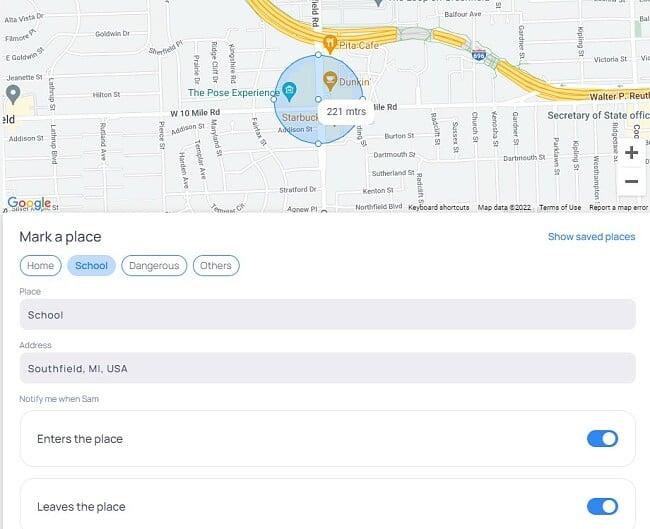The image showcases a computer monitor displaying Google Maps. The map interface includes a Marketplace section at the bottom and a "Show Saved Places" option to the right. Prominent tabs labeled "Home," "School," and "Dangerous" appear, with "School" being highlighted. 

Beneath these tabs, there's a search box with "School" entered, followed by an address box indicating "Southfield, Michigan, USA." Underneath, there’s a notification setting that reads "Notify Me When Sam," featuring two options: "Enters the Place" and "Leaves the Place," both toggled on to the right.

The map itself displays a circular area highlighting key locations such as a Dunkin' Donuts, Starbucks, and a place named "The Polls." It notes a distance of 221 meters within this highlighted circle. The interface consistently reiterates the tabs, place, and address information.

Overall, the map interface effectively tracks and notifies the user's whereabouts related to the "School" location in Southfield, Michigan.